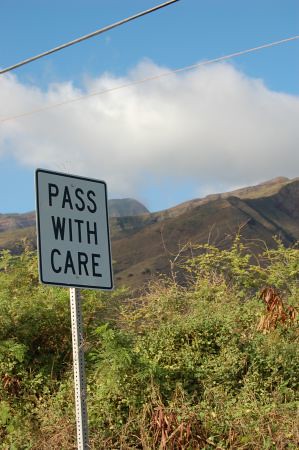The image depicts a "Pass With Care" road sign mounted on a typical perforated silver metal pole, taken from below looking upwards. The sign, featuring black letters on a white background, stands prominently in the foreground. Behind the sign, an unkempt area filled with green brush and dead leaves stretches out. Further back, rugged, brown mountain peaks rise, indicating a landscape devoid of snow. Above, a vivid blue sky stretches across the top of the image, punctuated by a large, fluffy white cloud. Cutting diagonally across this expanse are two telephone wires: one thicker and darker, running from the upper-left to the center-top of the image, and a thinner, lighter wire stretching from the upper-left to the upper-right.